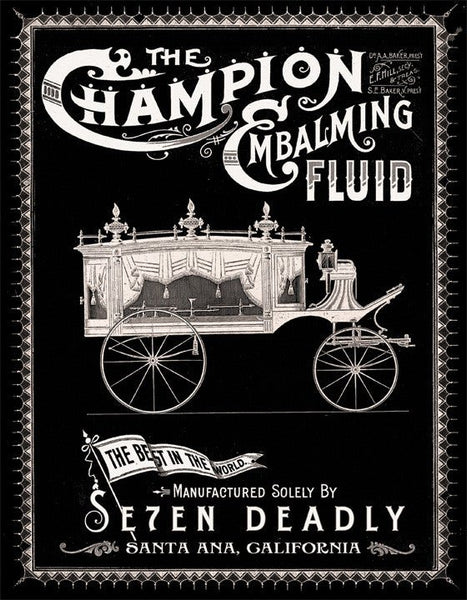This is a vintage black-and-white poster advertising "The Champion Embalming Fluid," showcasing intricate, ornate lettering. The poster features a striking zigzag white border with small detailed tufts. Dominating the center is an illustration of an old-fashioned horse-drawn hearse, resembling a royal coach, complete with a large rear wheel and smaller front wheel. The hearse has glass windows adorned with luxurious white curtains and tassels. Below the illustration, a flowing banner reads "The Best in the World," conveying a sense of movement in the wind. Further down in white lettering, it states the manufacturer: "Manufactured Solely by Seven Deadly," with the 'V' uniquely styled as a numeral '7', followed by "Santa Ana, California." This elaborate and richly detailed advertisement captures the essence of its era, blending functionality with an artistic touch.